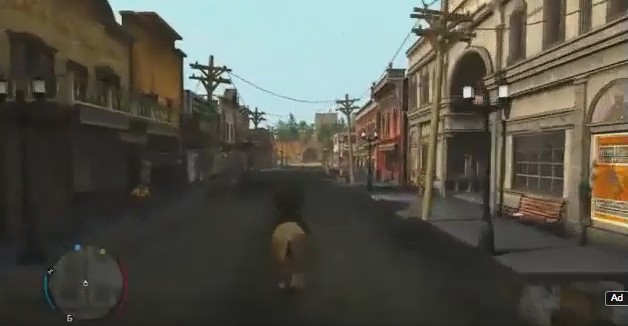This screenshot appears to be from a video game, capturing a somewhat blurred scene within a city setting. At the center, there's a character riding a beige-brown horse, dressed in all black attire. The scene is filled with two-story buildings, some showing white, brown, and tan hues, while others in the distance exhibit a modern pinkish color, reminiscent of architecture from the late 1800s to early 1900s. Metal telephone poles and a few lit streetlights are visible, adding to the urban atmosphere. To the left, slightly obscured and in the distance, stands another person. A lone bench is present near the center-right of the image, grounding the scene in its everyday urban environment. Trees are scattered in the distant background, adding a touch of greenery. The game interface includes a circular map at the bottom left corner and an "Add" button in the bottom right, hinting at some interactive elements.